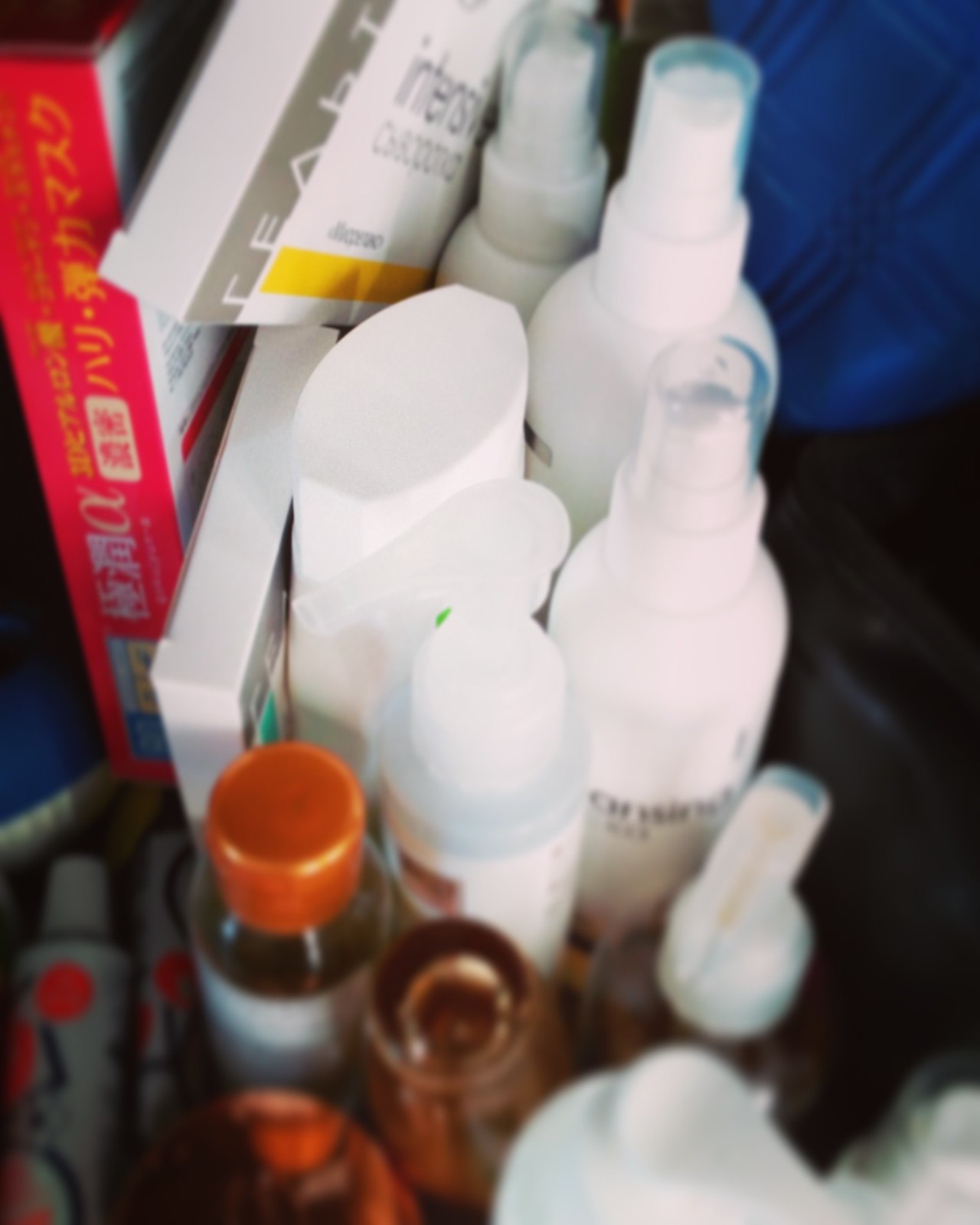In this color photograph, we observe the top of a cluttered shelf adorned with various items. In the upper left corner, a red textbook with Chinese characters stands upright, providing a striking contrast to the other items. Beside it, several books lie on their sides, though their titles are obscured. Moving rightward, three white pump spray bottles with clear lids are lined up neatly. Behind these spray bottles, a white shampoo bottle with its own pump is visible, partially concealing another shampoo bottle designed for pouring. 

Toward the top right corner, a blue blanket is discernible, adding a hint of color variation to the scene. The bottom left corner reveals a collection of tubes, possibly containing paste, alongside petite glass jars, one of which boasts an orange lid that unscrews for access. Nestled in the bottom right corner of the image, another spray bottle makes its appearance, completing the eclectic assortment of items. This detailed assembly provides a glimpse into a diverse array of personal care and household products meticulously arranged on a high shelf.